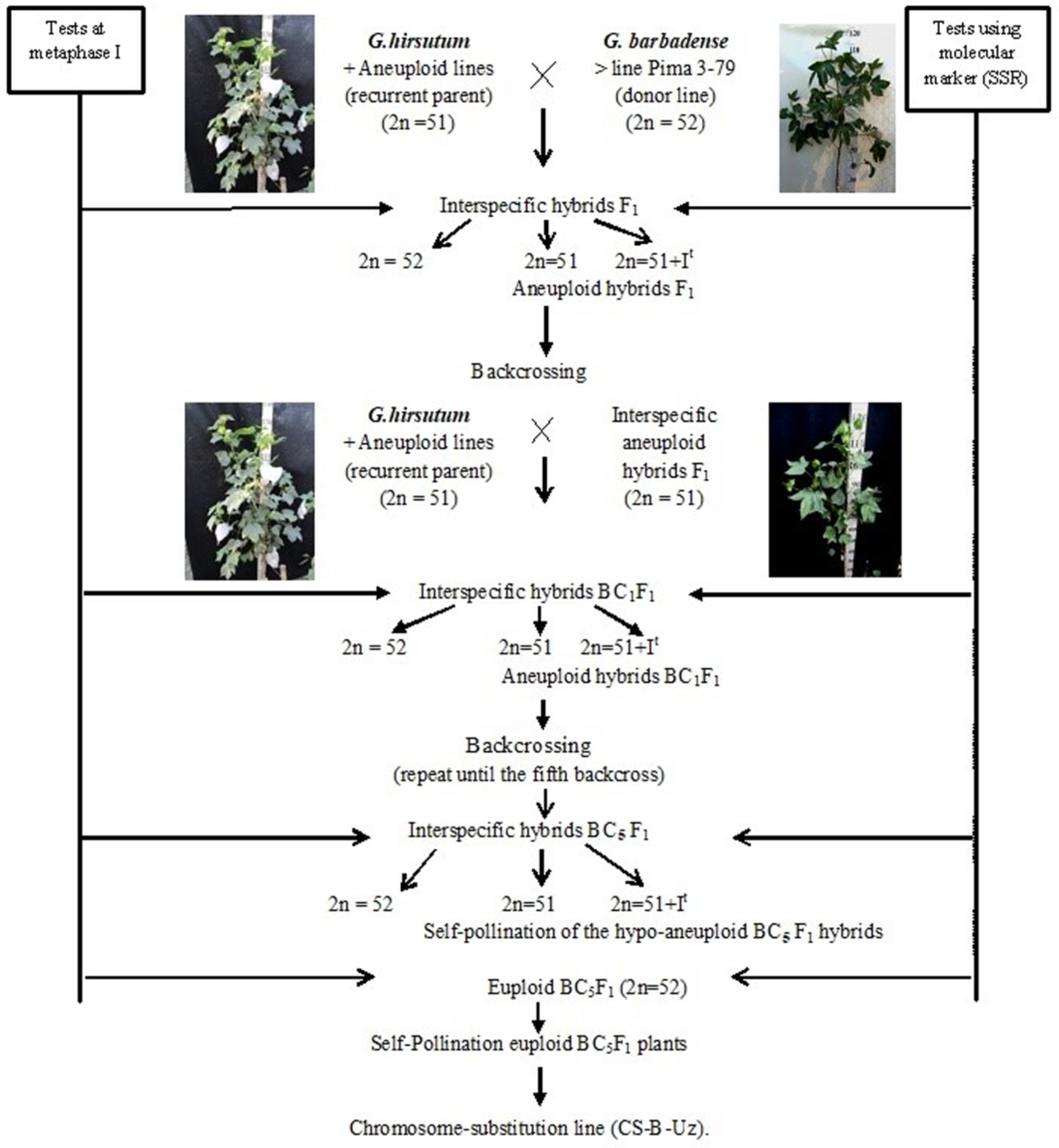The vertically aligned rectangular image features a detailed flowchart on a white background, bordered in black on the left and right sides. At the top left, it begins with "Test at Metaphase 1," alongside images of plants labeled "G. hirsutum" and "G. barbadense," with accompanying text: "G. hirsutum + aneuploid lines, recurrent parent, 2n = 51" and "G. barbadense, line Pima D379, donor line, 2n = 52." 

Arrows direct the viewer downwards and laterally, indicating a progression of experimental stages. The next section lists "Interspecific Hybrids F1," followed by down arrows leading to labels such as "Test using molecular marker SSR" and additional images of hybrid plants displaying characteristics like leaves and flowers. This is accompanied by more detailed information and genetic equations like "2n = 51" or "2n = 52."

The diagram further specifies "Interspecific Hybrids BC1 F1," with additional arrows pointing to the left and right, representing further crossing stages and genetic details. The progression continues through multiple backcrossing phases—BC2 to BC5—each stage illustrated with more plant images and genetic annotations.

Eventually, the chart presents "Self-Pollination of Hypoaneuploid BC5 F1 Hybrids" and "Self-Pollination Euploid BC5 F1 Plants," culminating in "Chromosome Substitution Line CSBUZ." Overall, this comprehensive diagram illustrates the experimental steps in crossing and backcrossing G. hirsutum and G. barbadense plant species, enriched with visual aids and detailed genetic information.